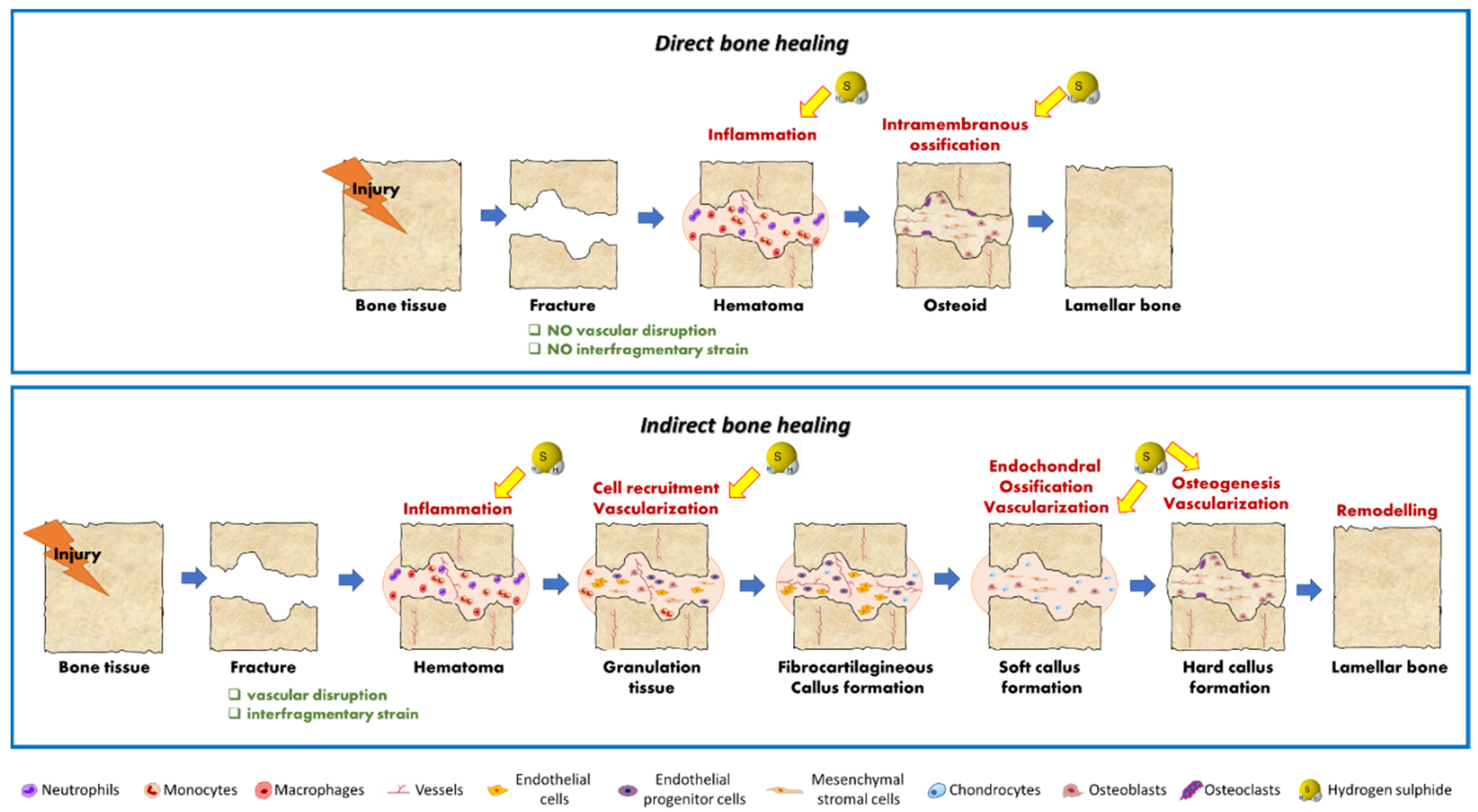This medical illustration showcases the detailed processes of direct and indirect bone healing in a clear side-by-side comparison within a white background framed by a thin blue border. The upper section, labeled "Direct Bone Healing" in black, italicized sans-serif font, provides a step-by-step visual sequence starting from the initial bone injury depicted by a lightning bolt hitting the bone, representing the fracture. Following this, the stages include inflammation and hematoma formation, visualized with a pink cloud and rippling red atoms, transitioning into osteoid formation (intramembranous ossification) with pink and purple dots amid a pink membrane. The final stage, lamellar bone formation, shows the bone fully healed with checkboxes indicating "no vascular disruption" and "no interfragmentary strain," though they remain unchecked.

The lower section, labeled "Indirect Bone Healing" in the same font style, also tracks the healing process but with more complexity, delineated in eight visual blocks. It begins similarly with bone tissue injury and fracture, followed by inflammation and hematoma, then progresses to cell recruitment, vascularization, and granulation tissue formation. This section continues through fibrocartilaginous callus formation and endochondral ossification, highlighting stages such as soft callus formation, vascularization, and hard callus formation before culminating in remodeled lamellar bone. Like the direct bone healing, the checkboxes for "vascular disruption" and "interfragmentary strain" are present but unchecked.

The diagram is enhanced with color-coded arrows and text to guide the viewer through each phase. A legend at the bottom clarifies various cell types involved in both processes, including neutrophils, monocytes, macrophages, endothelial cells, progenitor cells, mesenchymal stromal cells, chondrocytes, osteoblasts, osteoclasts, and a mention of hydrogen sulfide. This comprehensive depiction robustly elucidates the regenerative journey from bone injury to complete healing.